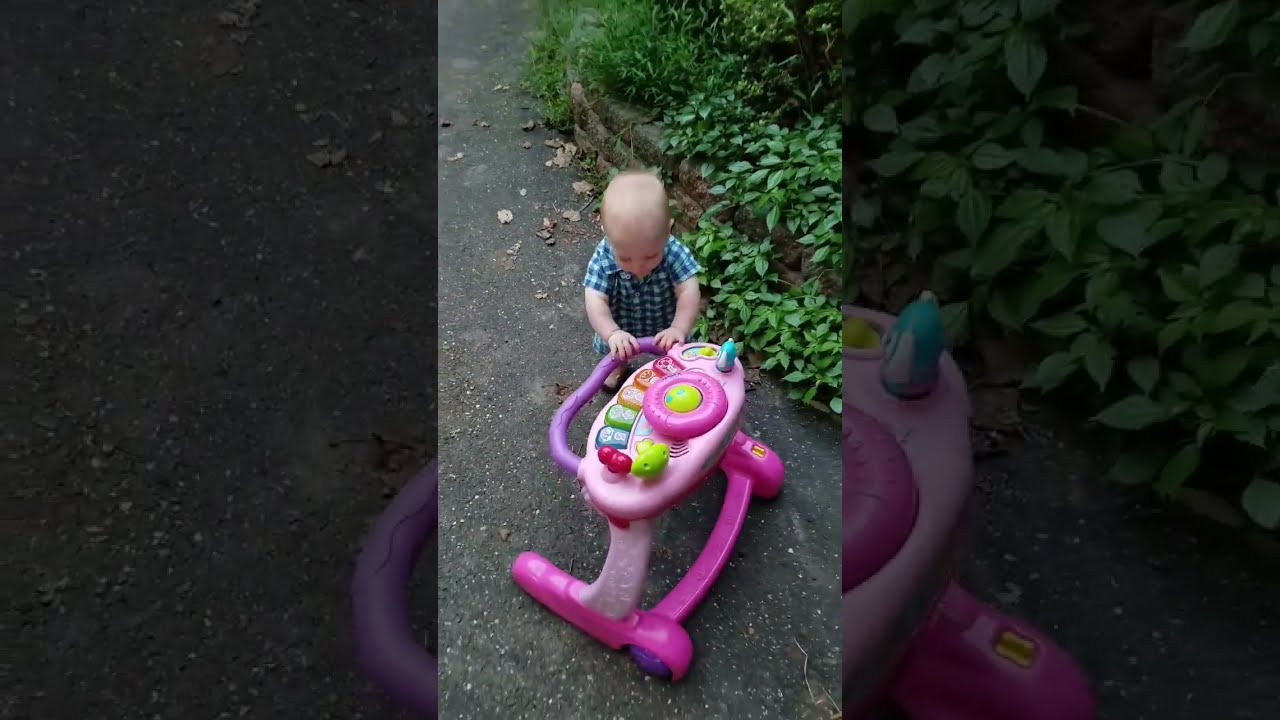In this color photograph set in a black background landscape orientation, a young blonde toddler, approximately 9 to 12 months old, is seen standing outdoors during the day. The child, dressed in a blue and white checkered one-piece outfit, is using a brightly colored toy walker for support. This toy features a pink base, purple plastic stand, and a circular top adorned with blue, green, orange, and red tabs, along with a pink donut-shaped piece with a blue center. The toddler is positioned next to the wheel of a red SUV, with a black SUV parked behind it. The scene unfolds on a sidewalk or driveway adjacent to a wooded area, visible in the upper right corner of the photo, where green trees and scattered brown leaves are seen on the forest floor.